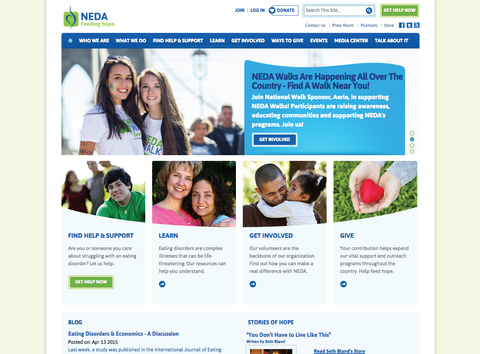**Detailed Description of the Image:**

At the top of the image, the background is white. In the top left corner, the text "NEDA feeding hope" is displayed, with "NEDA" in blue and "feeding hope" in green. Accompanying this text is a logo consisting of green and blue colors.

Standing out on the top right, there are several blue buttons labeled "Join," "Log In," and "Donate." Adjacent to these, there is a search box accompanied by a green button.

Continuing on the top right of the image, the text "Get Help Now" is prominently displayed.

Below this, a series of tabs are available, including "Contact Us," "Room," "Position," "Name," and icons linking to social media platforms such as Facebook, Twitter, and Reddit.

Further below, another set of tabs is visible near the bottom of the header, offering options like "Who We Are," "What We Do," "Find Help and Support," "Where to Give," "Events," "Health Centre," and "Talk About It."

The lower part of the image features several people wearing white t-shirts with "NEDA Talk" written on them. To the right, text explains that "NEDA works are happening all over the country" and encourages viewers to "Find a worker near you. Join national work sponsors early in supporting NEDA work. Participants are raising awareness, educating, communicating, and supporting NEDA's program. Join us." Additionally, there is a button labeled "Get Involved."

Following below are sections named "Find Help and Support," "Learn," "Get Involved," and "Give."

At the very bottom, there is a segment for the blog titled "Stories of Our Hopes," with the text "You don't have to live like this" in blue, along with the website of the blog.